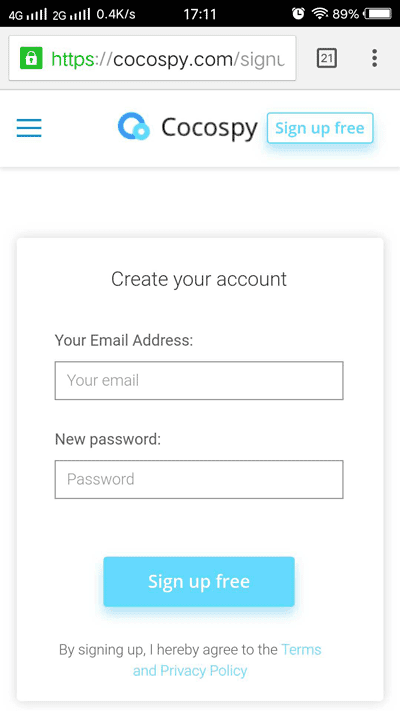This image showcases a webpage from CoCosby.com, featuring a clean and user-friendly sign-up interface. At the very top, the URL "CoCosby.com" is displayed, accompanied by a green HTTPS indicator and a white lock icon, signaling that the website is secure. Beneath this, there are three blue lines and a big blue circle with a light blue circle inside it, forming the CoCosby logo. 

Prominently displayed in black text are the words "CoCosby," followed by "Sign up free" written in blue within a white text box bordered by blue. Below this, a section labeled "Create your account" appears in a white text box with black text, prompting users to enter their email address and new password into corresponding fields.

Further down, a blue button with white text reads "Sign up free." At the bottom of the section, a disclaimer in black text reads, "By signing up I hereby agree to the," followed by blue, clickable links for "terms" and "privacy policy." The interface design maintains a cohesive black-and-white color scheme, with accents of blue for interactive elements and emphasis on the CoCosby brand.